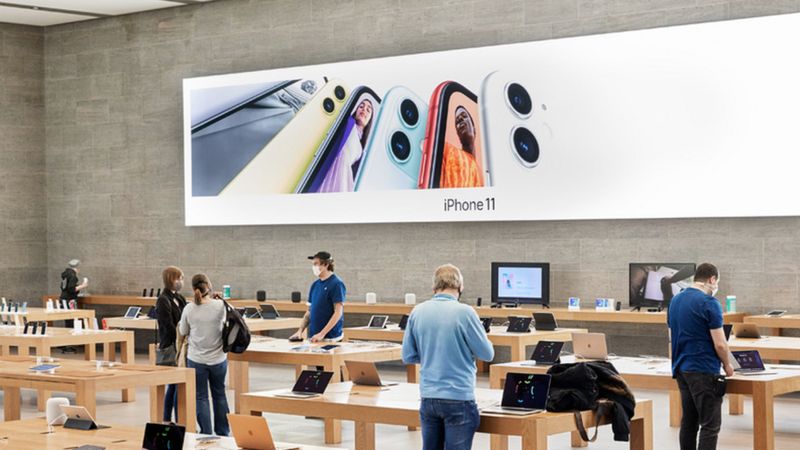The image depicts a modern Apple Store, characterized by its minimalist and industrial design. The store features numerous Scandinavian-style, sandalwood-colored tables arranged in an open layout, each displaying a variety of Apple products such as iPhones, iPads, and laptops. 

The walls are constructed to simulate a gray cinderblock look, contributing to the store's clean, modern aesthetic. A significant, eye-catching poster along one wall prominently advertises the iPhone 11, suggesting that the photo was taken approximately four years ago during the COVID-19 pandemic, as evidenced by the face masks worn by the people in the store.

The ceiling is a sleek white drop design, enhancing the bright and spacious feel. Around eight tables are visible, with about eight young individuals engaging with the displayed products, testing and exploring them in an uncrowded, relaxed atmosphere.

Despite the bustling activity, there are no chairs, underscoring the store's design for mobility and interaction. The scene captures a typical day in an Apple Store during the early release phase of the iPhone 11, reflecting modern retail design without any explicit promotional elements.